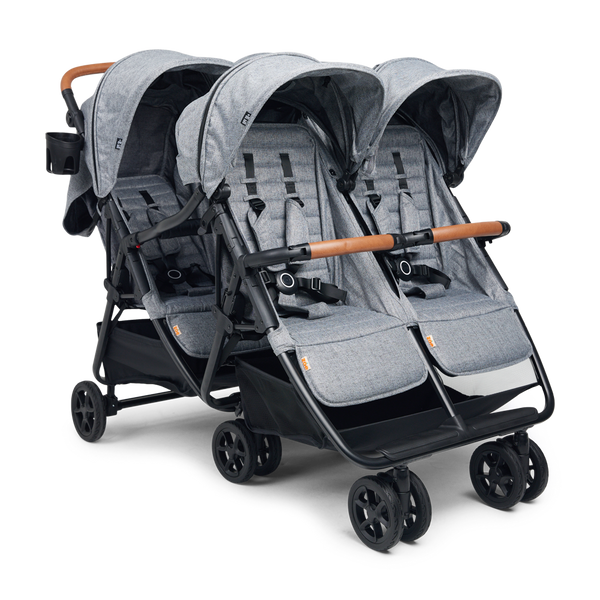The image features a professionally taken product photo of a quad stroller, set against a clean, white background. This sophisticated stroller is designed to accommodate four children, arranged in two rows of two seats each. The entire structure boasts a sturdy black metal frame with sleek black wheels. Notably, the stroller has three axles with the front and middle axles featuring double swivel wheels for enhanced maneuverability, while the rear axle has single wheels for stability.

Each seat is outfitted with a light and dark gray padded interior and includes individual sunshades that can be extended or retracted to shield the children from the sun. The front row of seats is equipped with a distinctive wood and black safety bar, reminiscent of a rollercoaster, which children can hold onto. Safety harnesses are also visible on the seats to securely buckle in the little passengers.

Underneath each row of seats, there are practical, flexible fabric storage baskets for carrying diaper bags or other necessities. The adult pushing the stroller can grip a stylish wood and black handle, which also incorporates a convenient black plastic cup holder on the left side. The overall design suggests a blend of functionality and elegance, tailored for families with multiple young children.